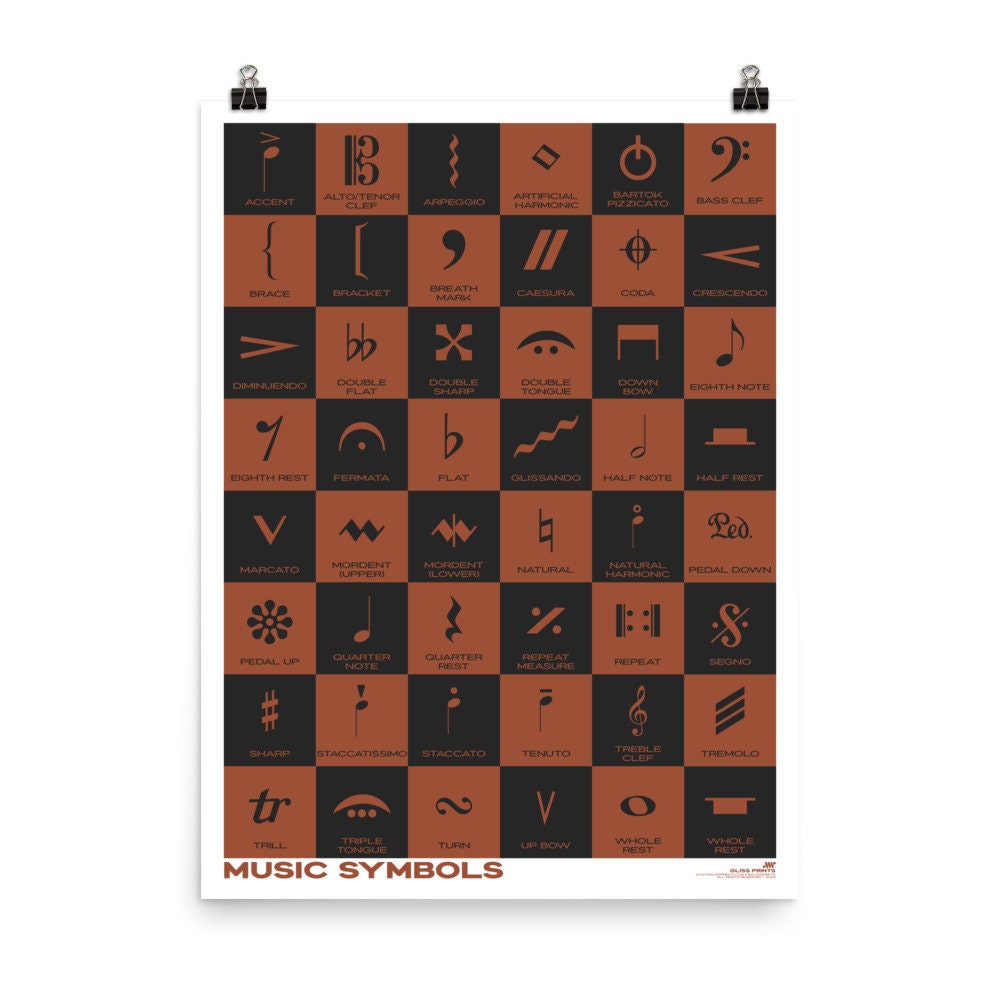The image is an informative sheet on different musical symbols, held up by two clips at the top corners of the paper. The sheet features a checkerboard pattern, alternating between red (or possibly orangey-brown) and black squares, each depicting a different musical symbol along with its name. Symbols such as accents, flats, half notes, half rests, double sharps, double flats, eighth notes, and breath marks are among the various symbols represented. The term "music symbols" is prominently displayed at the bottom left in a bold red color, further indicating the sheet’s educational purpose.